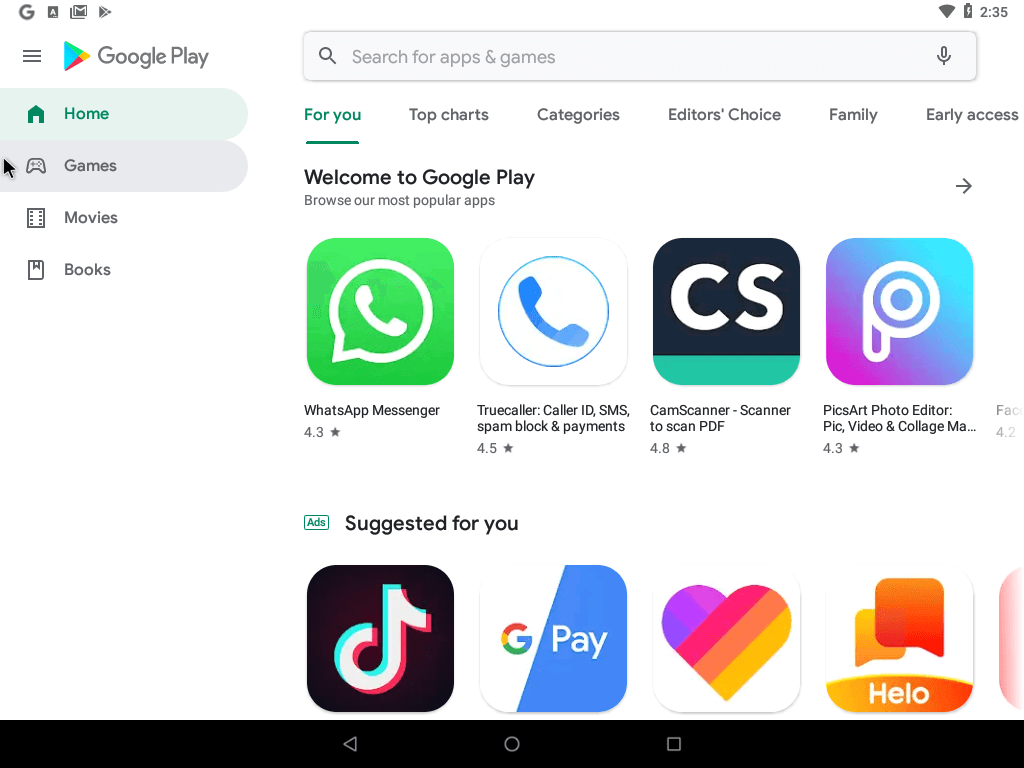The image showcases a tablet screen displaying the Google Play Store interface. The background is predominantly white, and at the bottom of the screen is a black navigation bar featuring the back button, home button (a circle), and the recents button (a square). The Play Store is currently on the home page under the "For You" category, with a welcome message prominently displayed.

In the main content area, there is a selection of app recommendations such as WhatsApp Messenger (green WhatsApp logo), Truecaller (caller ID, SMS, spam blocking, and payments), CamScanner, and PicsArt (blue and purple logo for the photo editor). Below these recommendations, there's a section for ads suggested for the user, including popular apps like TikTok and Google Pay. Several app logos are visible without accompanying names.

At the top of the screen, a search bar features a magnifying glass icon labeled "Search for apps and games," alongside a button for voice search. Menu options along the top allow for navigation to additional categories like "Games," "Movies," and "Books." The user’s mouse cursor highlights the "Games" section, indicating an imminent selection but confirming the current view is the home page.